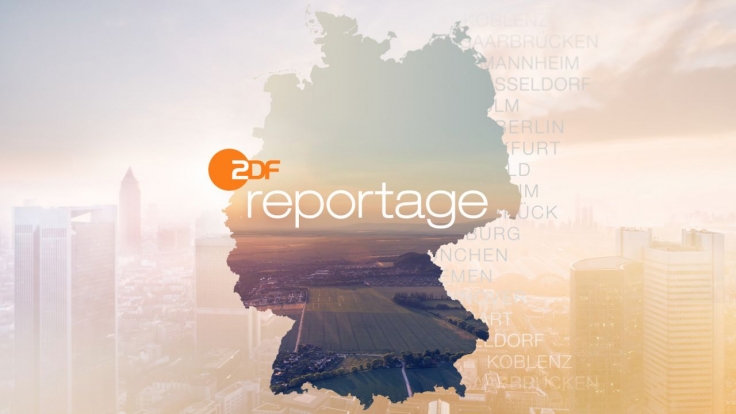In this image, a blurred cityscape stretches widely, showcasing tall buildings on both the left and right sides and even more structures fading into the distance. The city is bathed in a mix of pink, yellow, and gray hues, with some clouds adorning the upper right-hand corner. Dominating the center of this cityscape is a sharply contrasted cutout displaying vibrant fields of land divided into vertical strips, set against a darker gray sky with pink and white clouds. Central to the composition is the bold white text "2DF Reportage," while to its upper left, a small orange circle features a white number two and an orange "DF." This image, possibly intended for a website or advertisement, also includes partially visible city names in transparent lettering along its edges, hinting at a German metropolitan context.